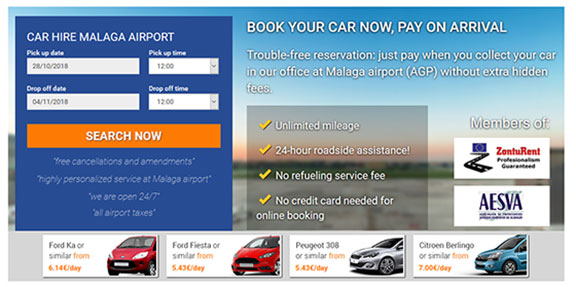The image is a detailed screenshot from a car rental advertisement at Malaga Airport. On the left side of the advertisement, the heading "Car Hire Malaga Airport" is prominently displayed. Below it, there are interactive sections for booking details: 

1. A text box labeled "Pick Up Date".
2. A corresponding drop-down menu for "Pick Up Time".
3. Similarly, fields for "Drop Off Date" and "Drop Off Time" are positioned beneath.

Beneath these fields, a prominent button states "Search Now". Additional text in this area advertises:
- Free cancellations and amendments
- Highly personalized service at Malaga Airport
- 24/7 operational availability
- Inclusion of all airport taxes

On the right side, a header says "Book Your Car Now". It provides several customer-friendly assurances:
- Payment only required upon arrival
- Trouble-free reservation process
- No extra hidden fees when collecting the car at Malaga Airport (AGP)
- Unlimited mileage for rentals
- 24-hour roadside assistance
- No refueling service fee
- No credit card needed for online booking

Below this section, affiliations with "Zontu Rent" and "AESVA" are mentioned.

Spanning the bottom of the ad, there are images of four different car models, each accompanied by their names and daily rental rates. This section provides a clear visual representation and pricing of available rental options.